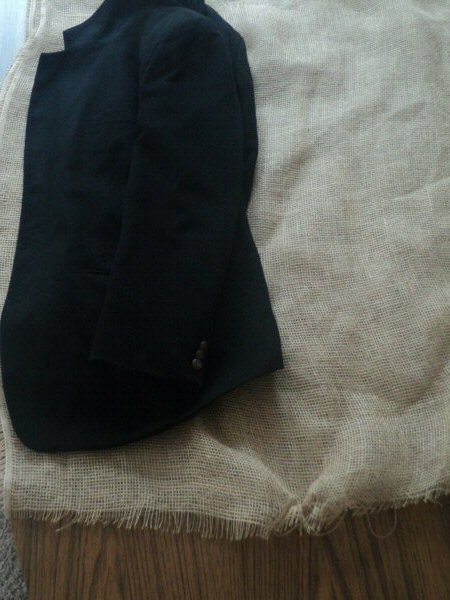The image shows a dark brown wooden surface with a distinct wood grain pattern that occupies the bottom section of the frame. Most of the area is covered by a large piece of light tan fabric, likely made of muslin or burlap, which appears thin and slightly fringed at the ends. The fabric is draped over the surface, creating the impression of a blanket or tablecloth. On top of this fabric lies a folded black suit jacket, primarily positioned towards the upper left side of the image. The jacket, which seems thick and could be made of wool or cotton, is folded in half with the sleeve prominently in view. There are three black buttons visible on the sleeve, giving it a formal appearance, potentially resembling a school uniform blazer. The overall lighting is slightly dim, adding to the subtle contrast between the black jacket and the tan fabric beneath it.